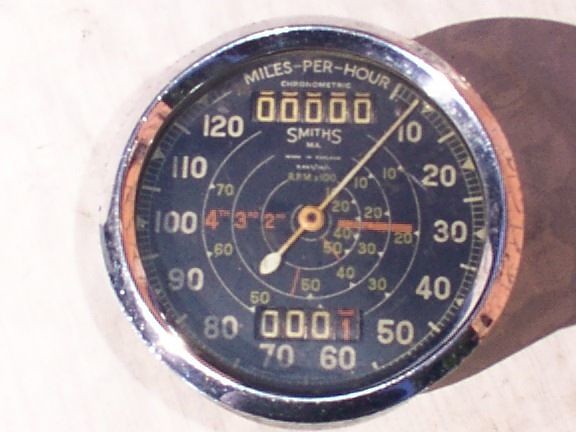The image features an antique odometer placed on its bottom edge against an off-white backdrop, casting a mid-tone brown shadow to the right. The outer rim of the odometer, constructed from chrome or possibly stainless steel, shows signs of pitting and rust, indicating its age and need for polishing. The face of the odometer is black, with "Miles Per Hour" inscribed in white across the top arc. The odometer reading shows 00000 in a rectangular window at the top, with a slight increment of one-tenth of a mile displayed. The needle points to number 4, denoting a speed of four miles per hour. The dial is marked in increments of 10, up to 120 miles per hour. Concentric white circles, resembling a bullseye, adorn the center of the dial, leading to its base.